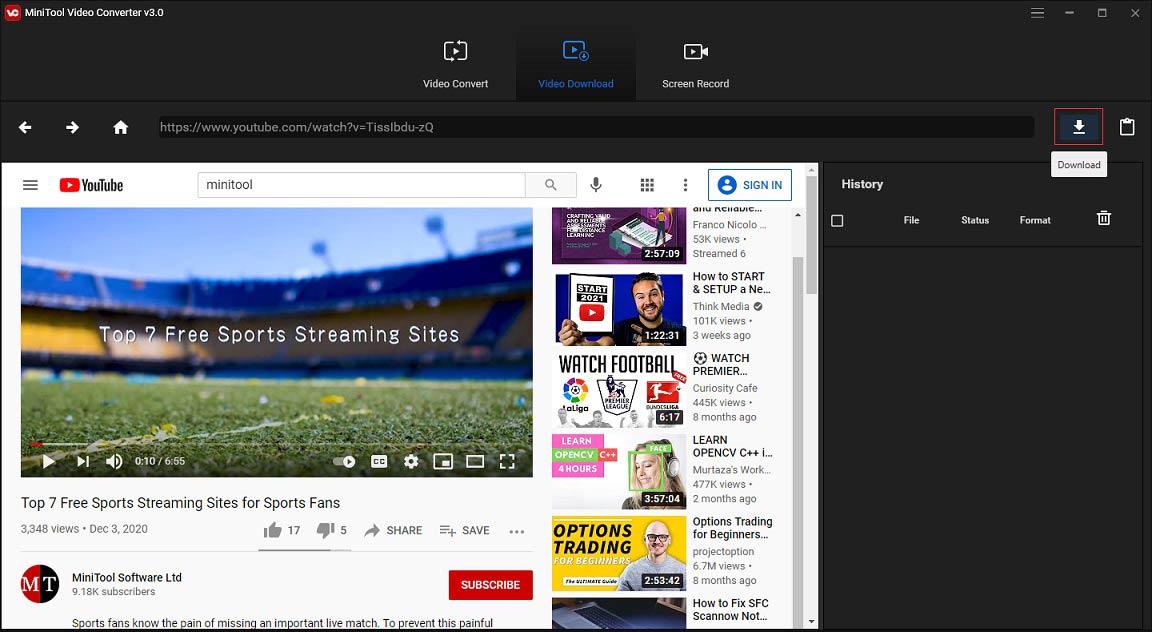This detailed screenshot depicts MiniTool Video Converter version 3.0, captured from a desktop or laptop. The application interface and background are black. At the very top, the menu bar displays the text "MiniTool Video Converter version 3.0" along with a small logo icon. On the same bar, to the right, are the minimize, full-screen, and close window icons.

Below the menu bar, three primary icons are visible: Video Convert, Video Download, and Screen Record. The Video Download option is selected, highlighted in blue while the others remain white. 

Directly beneath these icons is a search bar for entering video links. To the left of the search bar are three icons: a backward arrow, forward arrow, and a home icon. On the right side of the search bar are the download icon, highlighted in red with the text "Download," and the copy icon.

The main portion of the screen on the left is occupied by a small embedded YouTube window. This window is currently displaying a video titled "Top 7 Free Sports Streaming Sites for Sports Fans." Surrounding the video are suggested videos. Adjacent to this section is a sidebar labeled "History," which includes categories such as File, Status, Format, and a Delete icon at the bottom.